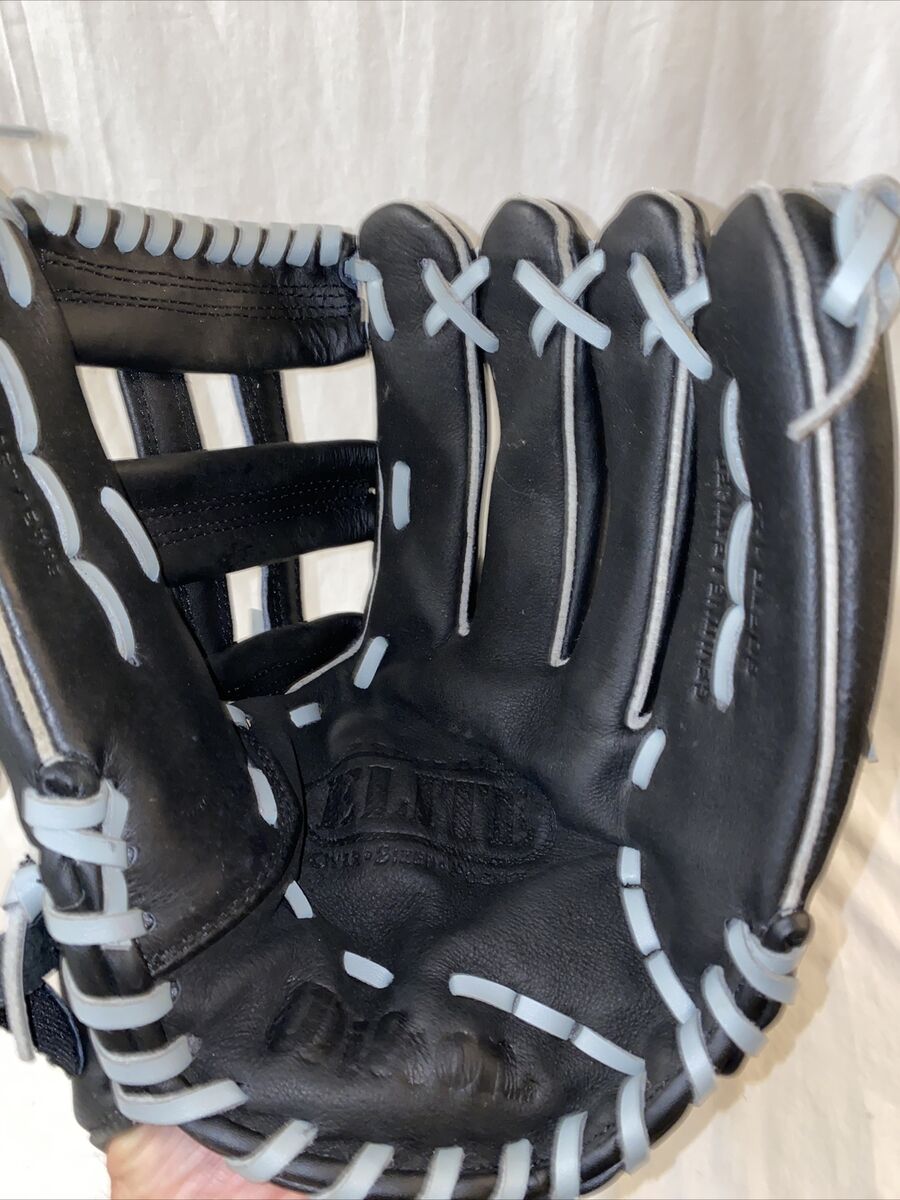This detailed close-up image captures the palm side of a black leather baseball mitt, specifically a left-handed mitt, against a white backdrop. The mitt features distinct white stitching, thick, flat gray leather strips, and three horizontal leather strips connected by two vertical strips between the thumb and the pointer finger, designed for catching balls. The glove is being worn by a person, with a tiny bit of their wrist visible at the bottom of the image, indicating it is worn by a Caucasian hand. The bottom edge of the glove showcases the "Wilson" logo, imprinted in black cursive on black leather, while the center of the palm displays the word "Elite," encircled by a printed design.